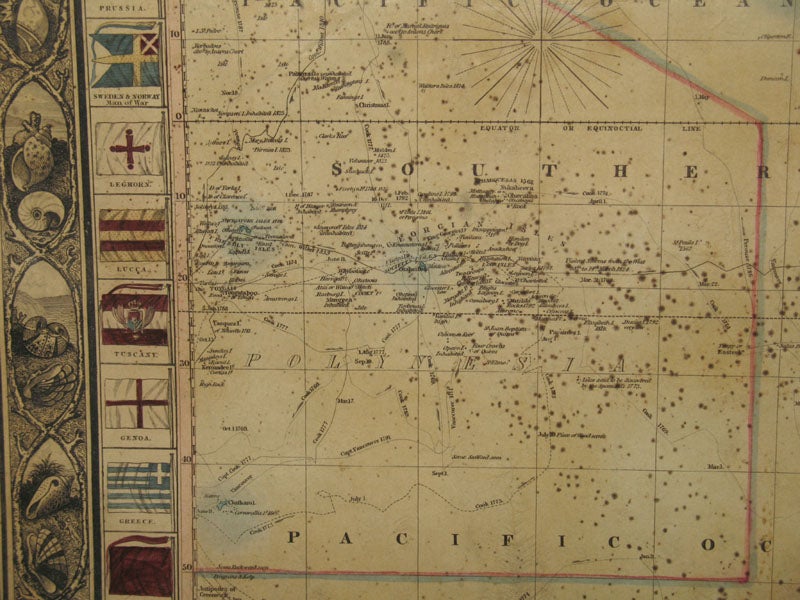The image depicts an ancient-looking map of the Southern Pacific region, presented in a landscape orientation. The map, with a grayscale base, is adorned with numerous tiny dots indicating various locations and geographical features. Running vertically along the left-hand side, a decorative border showcases hand-drawn seashells beside a series of flags, which seem to represent different countries or regions, including Sweden, Norway, Greece, Genoa, Lucca, Tuscany, and regions labeled Le Chur and Lucia. Notable labels on the map include "Southern Pacific," with the word "Ocean" abbreviated as "O.C." and partially cut off at the top, and "Polynesia" marked prominently in a lighter font. Despite the map's aged and damaged condition, which includes numerous black spots and difficult-to-read text due to its small size, you can discern latitude and longitude lines and spot several small islands within the indicated area. The map's overall design remains clean and meticulously detailed despite the wear.